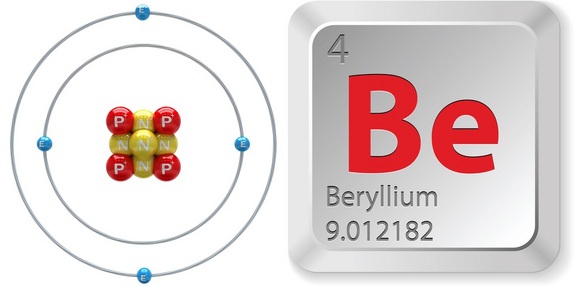This is an intricate illustration depicting the atomic structure and periodic table representation of the element beryllium. On the right side of the image is a shiny, silver-toned square, resembling a button or key, featuring the atomic number 4 in the upper left corner. Prominently displayed in the center are the large red letters "Be," with "beryllium" engraved beneath, followed by its atomic mass, 9.012182.

To the left, we see a detailed 3D model of a beryllium atom. At its core, there are four bright red spheres labeled with a white "P," representing protons, arranged in a square. Interspersed between the protons are five gold spheres marked with a white "N," denoting neutrons, with one neutron at the center of the square. Surrounding this nucleus are two orbital rings. The inner ring has two blue spheres labeled "e" on the left and right sides, indicating electrons. The outer ring also has two blue "e" spheres, positioned at the top and bottom. The entire design crisply displays the beryllium element's atomic structure, combining visual appeal with scientific accuracy.